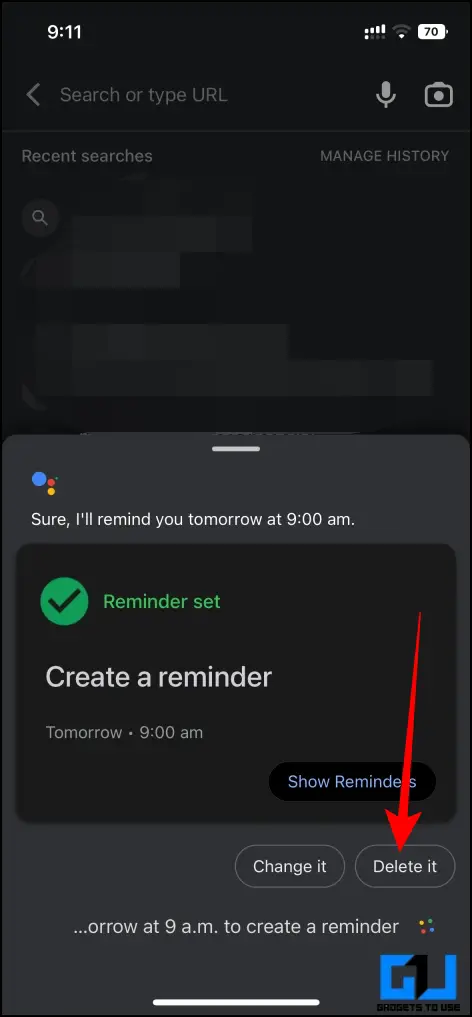In this screenshot, we observe a pop-up notification at the bottom of the screen that reads, "Sure, I'll remind you tomorrow at 9 a.m." and "Reminder Set." It indicates the creation of a reminder for 9 a.m. the following day. Below this message, there is a button labeled "Show Reminders." Additionally, two buttons are positioned beneath this section: one labeled "Change it" and the other labeled "Delete it." The text near the bottom appears to be partially obscured or colored over, showing only the fragment "O-R-R-O-W at 9 a.m. to create a reminder." A logo is present in the bottom right corner of the image, and "Gadgets to Use" is displayed at the top of the screenshot. In the upper left corner, the time is noted as 9:11, and the phone’s battery level is at 70%. A red arrow has been added to the screenshot, pointing downward towards the "Delete it" button and positioned next to the "Change it" button.